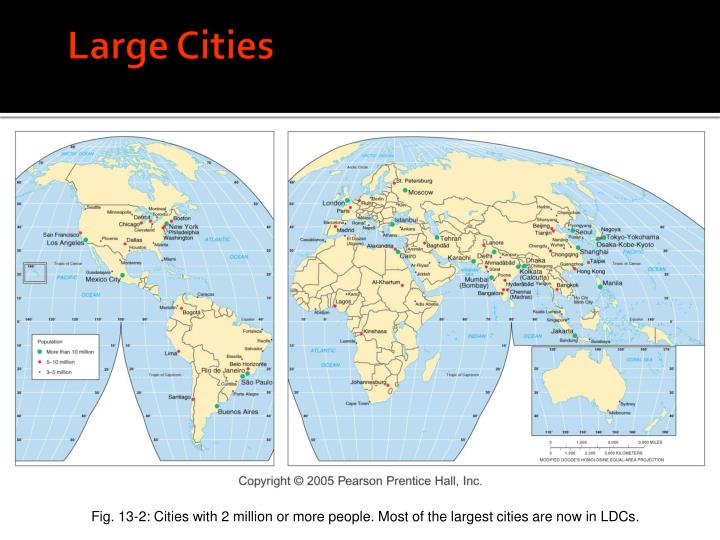This image is a detailed, textbook-style projection map of the Earth, divided into two adjacent hemispheres. The left side features the Western Hemisphere, showcasing North, Central, and South America with major cities such as Los Angeles, Mexico City, Washington, New York, Philadelphia, Lima, Buenos Aires, and Rio de Janeiro prominently labeled. The right side displays the Eastern Hemisphere, including Europe, Africa, and Asia, with notable cities like Moscow, Tehran, Johannesburg, Shanghai, Hong Kong, and Mumbai marked.

The Earth's surface is mapped with light blue representing water bodies and a light yellow or khaki color denoting landmasses. Latitude and longitude lines are clearly labeled, and country borders are delineated in black lines. Major cities are indicated with dots of varying colors based on population size: green for those exceeding 10 million, red for populations between 5 and 10 million, and brown for cities with 3 to 5 million residents.

Dominating the top fifth of the image is a horizontal black bar with the text "Large Cities" in red, capitalized letters. Below the maps, a caption reads "copyright 2005, Pearson, Prentice Hall, Incorporated. Figure 13.2, cities with 2 million or more people, most of the largest cities are now in LDCs," referencing that most large cities are currently in less developed countries.